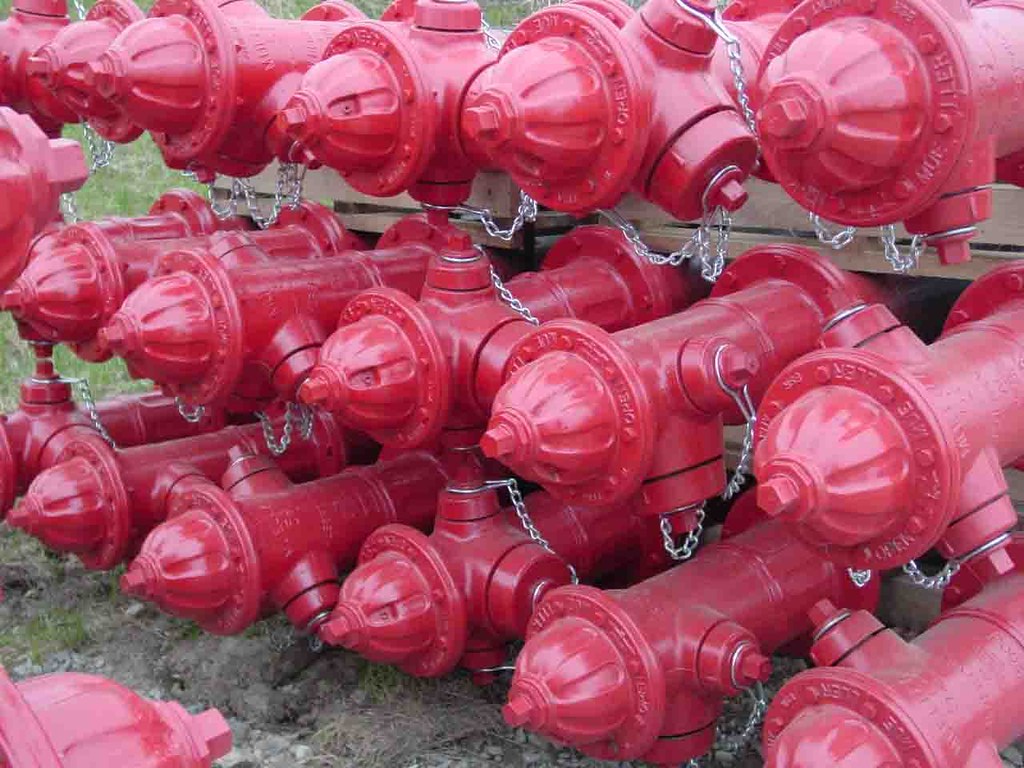In the image, numerous bright red fire hydrants are displayed, laying sideways in neat rows on a wooden rack. This rack, which supports the hydrants by their bases, is positioned on a surface that appears to be a mix of dirt and grass. Each hydrant is connected by a silver chain to the side caps where hoses would typically attach. There are three distinct rows, each containing about five or six hydrants. In the bottom left corner, a couple more hydrants can be seen, suggesting another similar wooden rack nearby. The scene takes place outdoors, presumably during the daytime, and the ground underneath the hydrants seems to be slightly concave.